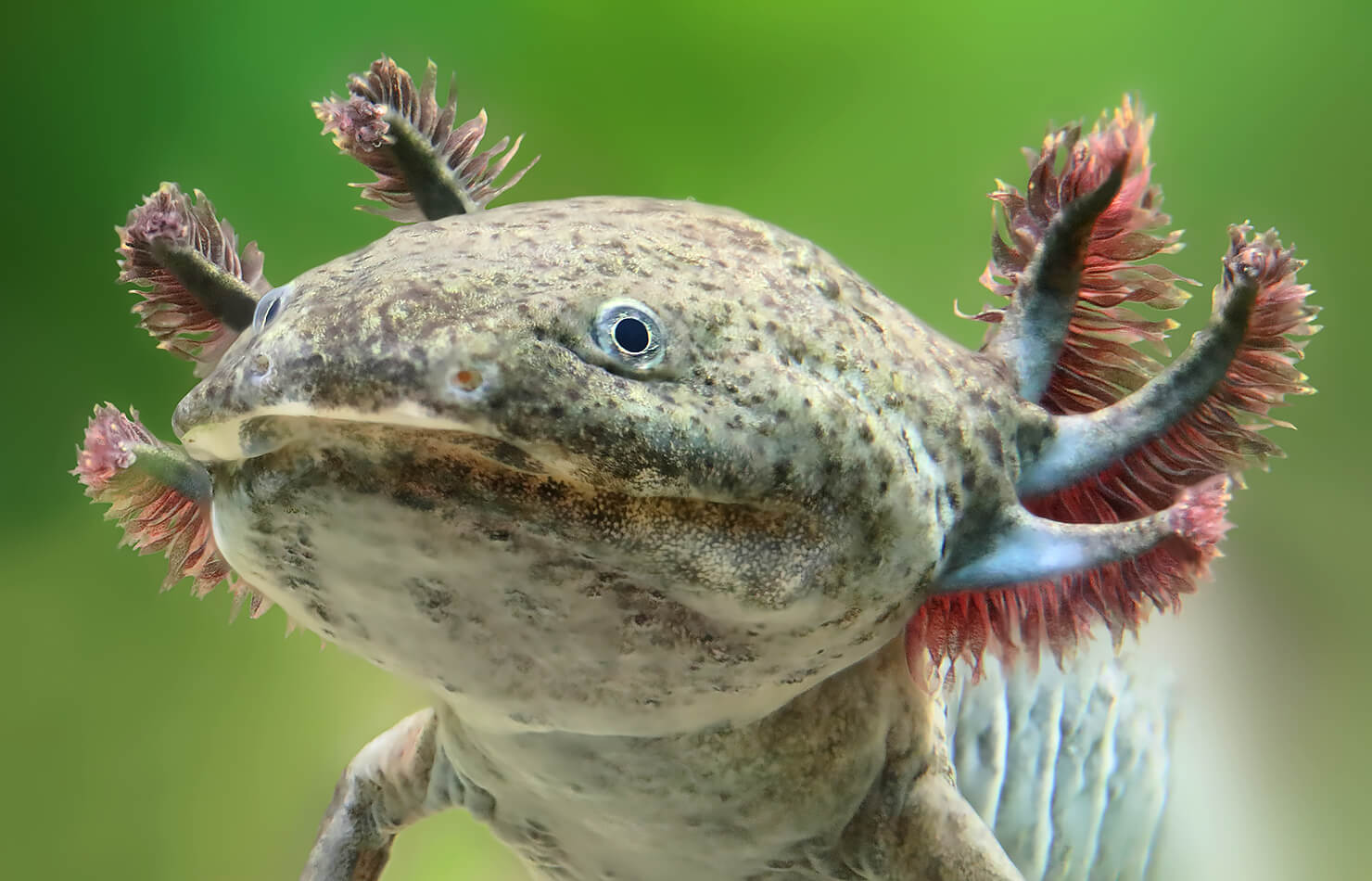This detailed color photograph showcases a close-up of an axolotl, a Mexican amphibious creature, set against a blurred green underwater background. The axolotl's large, rounded head is beige with darker speckles and bumpy textures, giving it a somewhat sandy and possibly moldy appearance. Its small, beady eyes are perfectly round, whitish on the outside with black pupils. The axolotl's head prominently features three horn-like protuberances on each side, adorned with dozens of red, spiny tentacles. The creature's wide-set, thin limbs are partially visible, and its mouth, though large, is closed. The image centers on the axolotl's face and head, allowing the unique details and vivid colors to stand out against the indistinct backdrop.